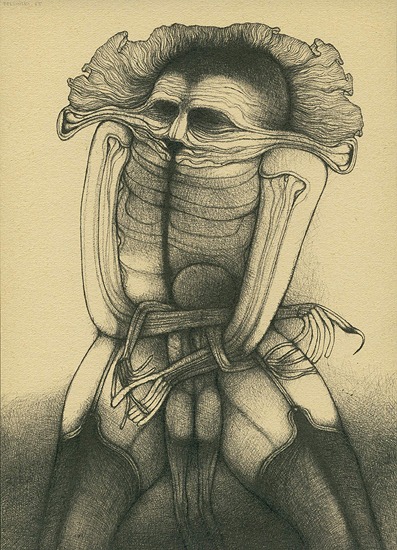This eerie, hand-drawn artwork, set against an off-white background that shades into gray towards the bottom, depicts a disturbing humanoid creature centrally positioned in the image. The figure has a small, distorted head that appears scrunched into its shoulders, with a face featuring grotesquely stretched eyes and mouth, creating a nightmarish expression. The creature's elongated, skeletal arms and fingers, which are entangled and bony in appearance, clasp a smaller, child-like version of itself between its stomach and thighs. This smaller figure could be mistaken for an additional set of legs upon first glance. The humanoid appears to be wearing high, metallic-looking stockings or armor that cover its thighs, adding to its unsettling appearance. The entire piece is rendered in shades of tan, black, and varying grays, emphasizing its creepy, horror-movie aesthetic. The background transitions from light cream at the top to dark gray at the bottom, intensifying the ominous atmosphere of the piece. This work, which seems to belong to a personal portfolio, showcases a high degree of detail and darkness, resembling a meticulous sketch with unsettling, macabre undertones.